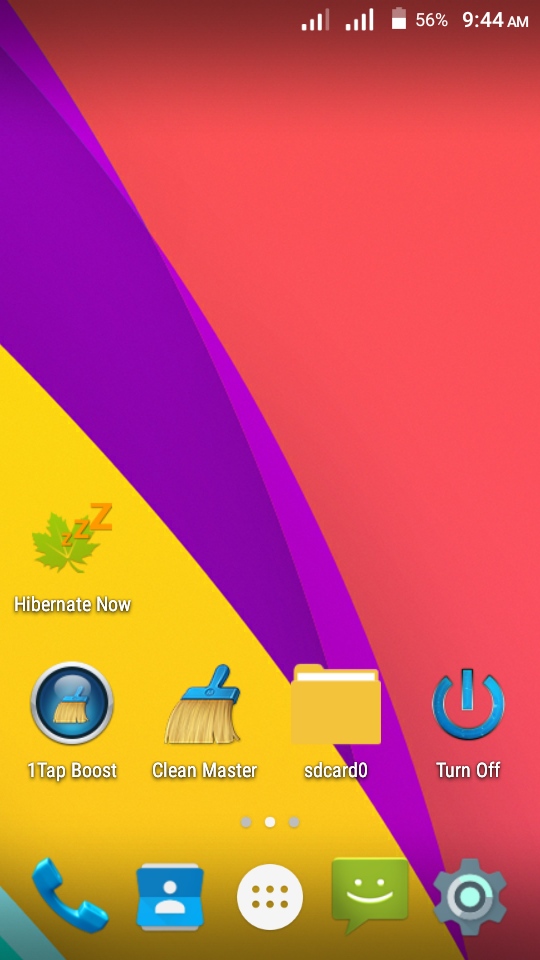This image captures a vibrant computer screen displaying various utility categories, each marked with distinctive visuals and text. The screen is divided into visually striking sections, featuring a predominance of red color covering the upper right corner down to the bottom right, and extending from the upper left to the bottom. A dynamic diagonal swath of blue cuts through the center of the screen, moving from the upper left to the lower right. Another triangular section of yellow sits beneath this blue swath, while the bottom left corner also hosts a blue triangle.

The on-screen categories listed include:

1. **Hibernate Now**: This category is represented by a symbol resembling a marijuana leaf, accompanied by three orange "Z's" emanating from it, indicative of sleep mode.
2. **One Tap Boost**: The icon here appears to be a blue mushroom-shaped cleaning brush with white bristles.
3. **Clean Master**: Illustrated by a small hand broom with a blue handle and yellow bristles.
4. **SD Card Zero**: Depicted by a yellow folder containing white papers visible at the top.
5. **Turn Off**: Marked by a blue power symbol within a circle.

All categories are labeled with white text, providing clear and readable labels against the colorful background.